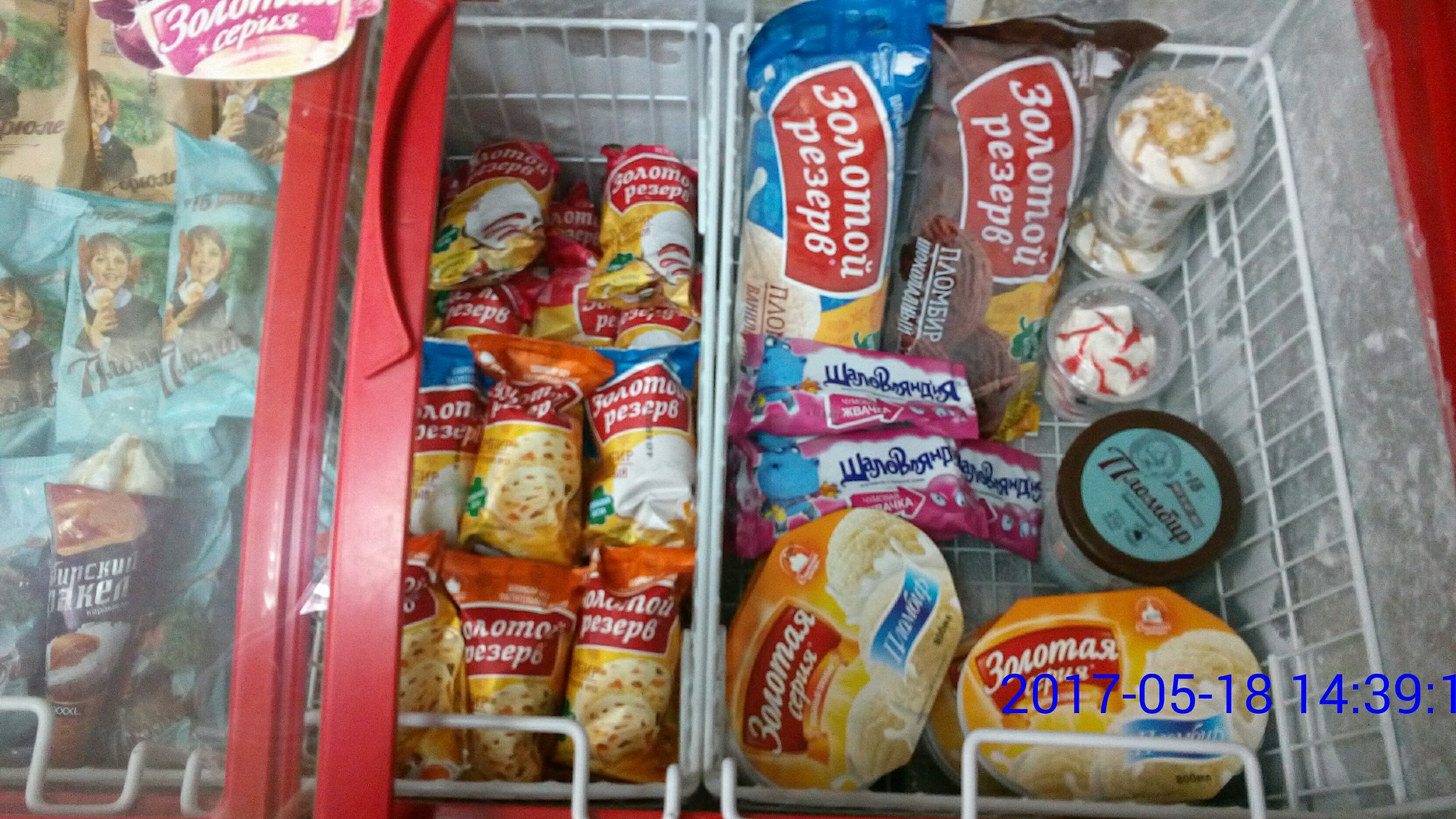A realistic photograph captures the interior of a horizontal chest freezer typically found in grocery stores. This low, ground-level cooler, about 2 to 3 feet tall, features a transparent top with a red sliding frame. The interior, made of stainless steel with white wire baskets, contains a variety of ice cream products and frozen treats packaged in yellow, blue, and brown wrappers. Some packaging features images of smiling women, while others display text in an unidentified foreign language. The bottom right corner of the image shows a timestamp in blue text: 2017-05-18 14:39:01.